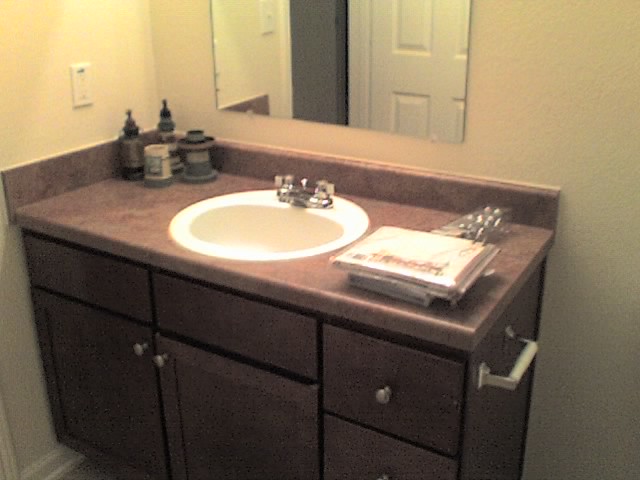A detailed photograph of a home bathroom sink, taken in a rectangular frame with longer top and bottom sides. In the center of the image, a dark brown wooden bathroom counter with matching dark brown veneer, mimicking stone, stands out. The counter features dark brown doors and drawers, each adorned with a silver-colored metal knob. On the right side of the counter, an empty toilet paper holder with a plastic rod is visible. Atop the counter sits a plastic bag containing metal items, and a shower curtain still sealed in rectangular plastic packaging. The wall behind the counter is painted white, complemented by a small rectangular mirror above the sink. The white sink below the mirror is equipped with a modest, metal silver faucet, flanked by two clear plastic knobs. The mirror reflects an open white door set in a matching white doorframe.